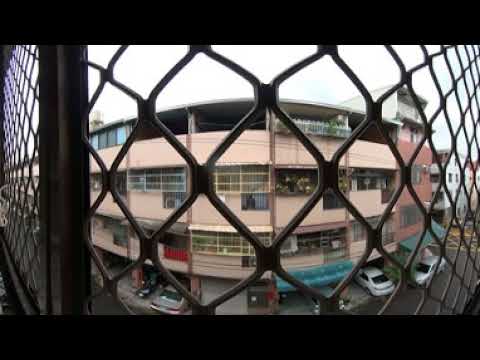This image captures a three-story, predominantly tan and pinkish apartment building as seen through a chain link fence with a distinct fisheye distortion. The building's facade features yellowish windows and multiple awnings: a blue one and a green one on the ground floor. Under these awnings, cars are parked, including a white car under the blue awning, a silver sedan under the green awning, and a tan sedan to the left of the center. The flat-roofed structure is surrounded by gray pavement, and the bright daylight illuminates details such as plants on the balconies. In the background, there's another white building partially visible. The sky above is a mix of whitish and light blue hues. The majority of the view is dominated by the chain link fence, which wraps around the image, and black borders appear at the top and bottom of the scene.